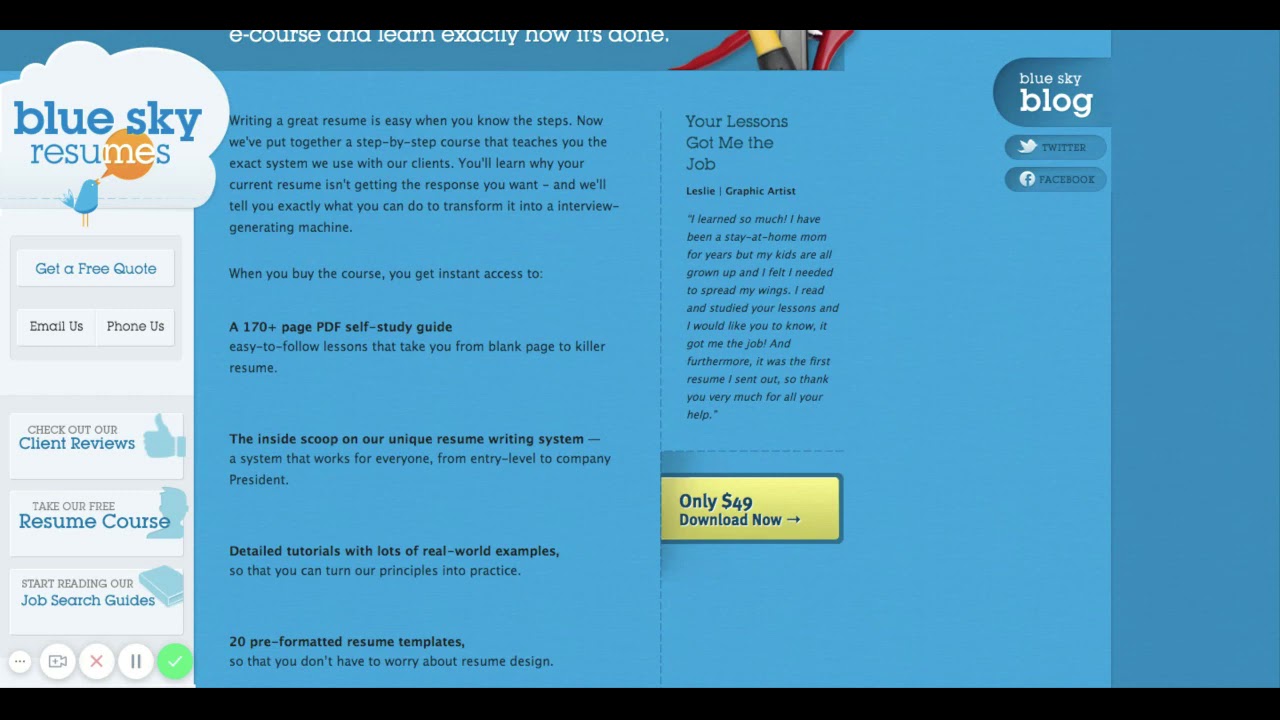The screenshot showcases the homepage of Blue Sky Resumes, a professional resume-building service. 

In the upper-left corner of the page, the Blue Sky Resumes logo is prominently displayed. The logo features the text "Blue Sky Resumes" within a cloud-like design. The words "Blue Sky" are written in blue letters, while "Resumes" is written in a combination of blue and white letters. Below this, there is an illustration of a blue bird with an orange speech bubble extending from its beak. The letters "ME" of "Resumes" are nested inside this speech bubble.

The main background of the webpage is blue, with sections of black text spread throughout the page. On the left side of the page, there is a white sidebar containing several navigational buttons. At the top of the sidebar, there's a button labeled "Get a Free Quote." Below it, there are two more buttons labeled "Email Us" and "Phone Us." Further down, there's a button that reads "Check Out Our Client Reviews," followed by another button that instructs visitors to "Take Our Resume Course." At the bottom of the sidebar, there's a link inviting users to "Start Reading Our Job Search Guide."

The central section of the webpage features a large yellow button, roughly in the center, that reads "Only $49, Download Now," accompanied by an arrow pointing to the right, indicating that this is the primary call-to-action for downloading their services.

In the upper-right corner of the webpage, there are several small bubbles for additional navigation. One bubble is labeled "Blue Sky Blog," and next to it are links to Blue Sky Resumes' Twitter and Facebook pages.

Overall, the webpage offers various tools and resources aimed at helping users create, improve, and manage their resumes and job search strategies.